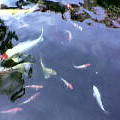This image depicts a small, square photo of a koi pond, taken from above as if the viewer is looking down into the water. The pond is partially obscured by the small size of the image, making some details challenging to discern clearly. Despite this, one can observe approximately eight to ten fish, mostly koi, swimming in the blue-tinted water. The fish are mainly white with some displaying orange or pinkish-red markings, particularly on their heads. Notably, there is one large koi fish with a white body and an orange head, contrasted by several smaller koi with similar white bodies and orange heads. The water itself appears somewhat opaque but calm, with the edges of the pond featuring rocky terrain interspersed with what looks like moss or seaweed. The overall scene suggests a tranquil and meticulously maintained aquatic environment.